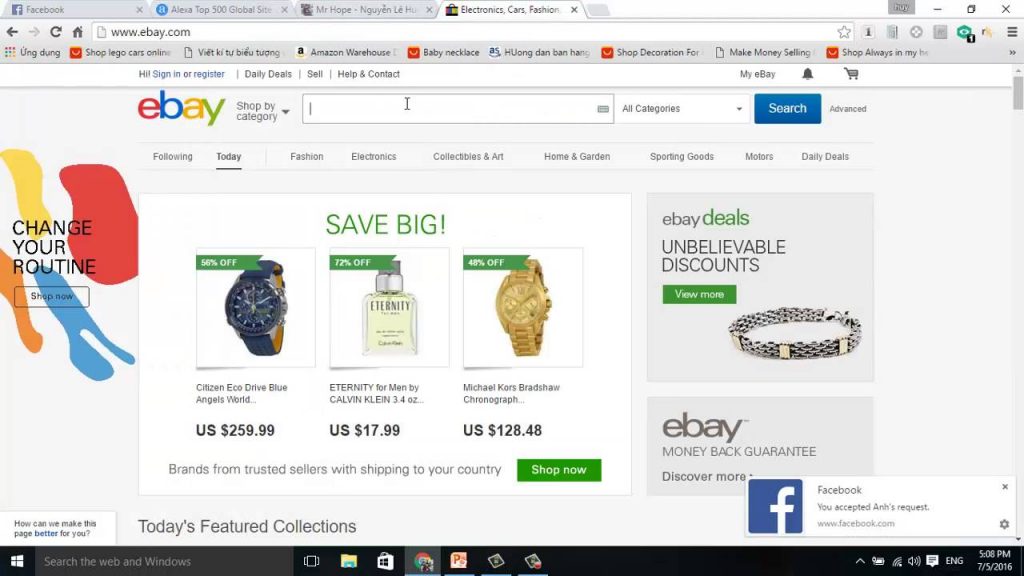This is a detailed screenshot of the eBay website homepage. Prominently placed in the upper left-hand corner is the iconic eBay logo, accompanied by a "Shop by category" text. To the right of this, a search bar is situated, followed sequentially by an "All Categories" drop-down menu, a blue "Search" button, and an "Advanced" search link.

Beneath the primary navigation area, a horizontal menu offers various categories: "Following," "Today," "Fashion," "Electronics," "Collectibles & Art," "Home & Garden," "Sporting Goods," "Motors," and "Daily Deals."

Below these menu items, vibrant green text urges visitors to "Save Big," next to images of highlighted products. Displayed are a blue watch priced at $259.99 USD, "Eternity" cologne by Calvin Klein for $17.99 USD, and a gold watch listed at $128.48 USD. The promotional text "Brands from trusted sellers with shipping to your country" lies beneath the products, accompanied by a green "Shop now" button.

To the right, there are several feature modules with light gray backgrounds. These highlight "eBay Deals," emphasizing "unbelievable discounts" with a green "View more" button. A silver bracelet image is also included. Finally, at the bottom, the eBay logo is repeated in gray, along with the words "Money Back Guarantee" and the invitation to "Discover more."